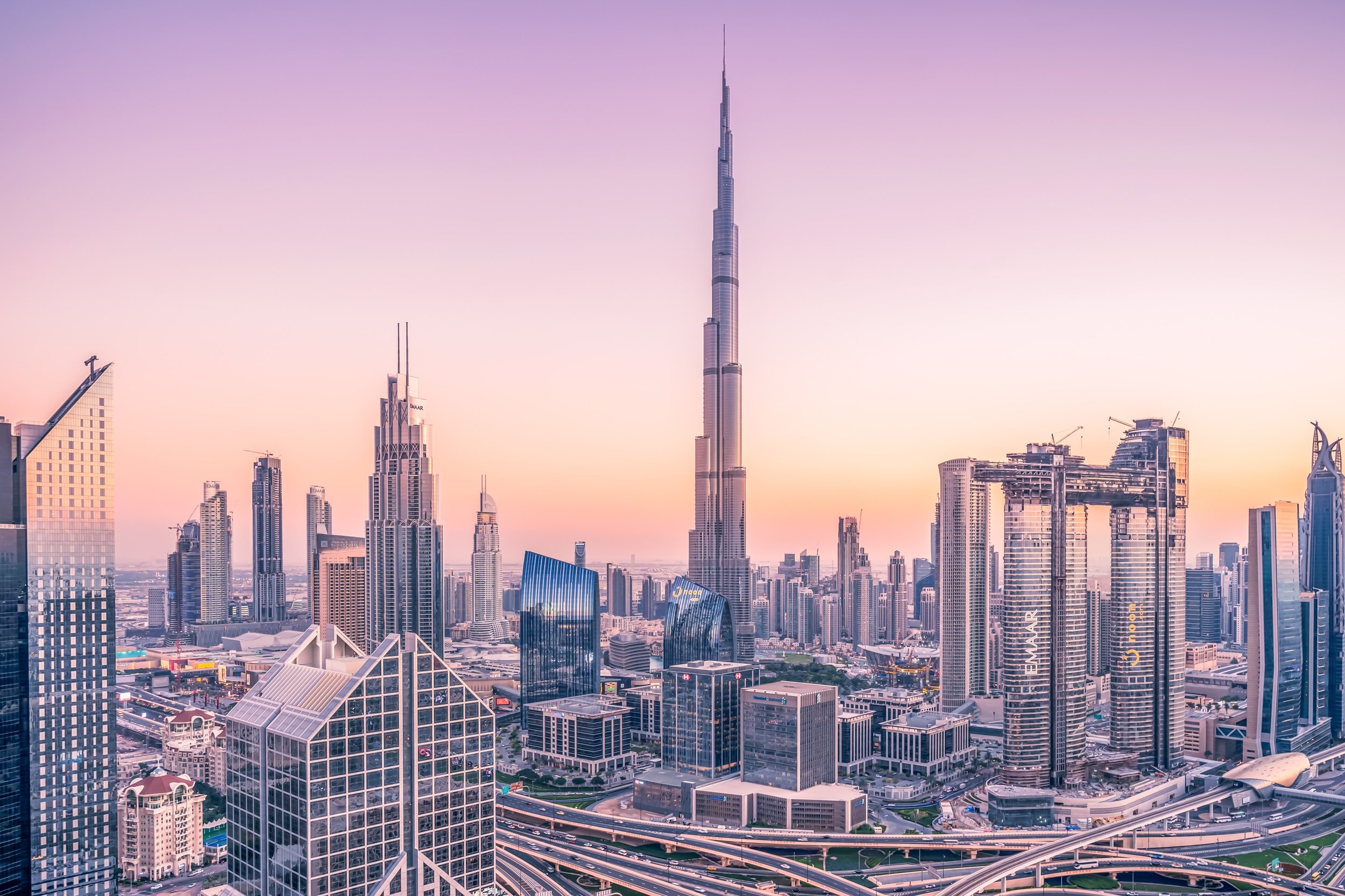This is an aerial view of a modern cityscape characterized by a plethora of tall, contemporary buildings with mirrored and shiny glass facades. The image depicts a bustling downtown area with roads intersecting on multiple levels and cars navigating the highways that loop and stretch in every direction. Dominating the center of the photo is a striking skyscraper with a needle-like spire reaching skyward, emphasizing the verticality of the scene. Surrounding this central structure are numerous other buildings, some with distinctive triangular and angled rooftops, including an A-frame design and a super thin building tapering to a near point with an antenna-like structure on top. The bottom right of the picture reveals the tops of various buildings, enhancing the complexity of the urban landscape. The scene is tinged with a vibrant pinkish hue, and the sky transitions from purple to shades of yellow, pink, and orange, suggesting an early morning or dusk setting. Adding to the modern ambiance, several billboards and written advertisements are visible in the background, and a domed modern train station can be discerned among the architectural ensemble.